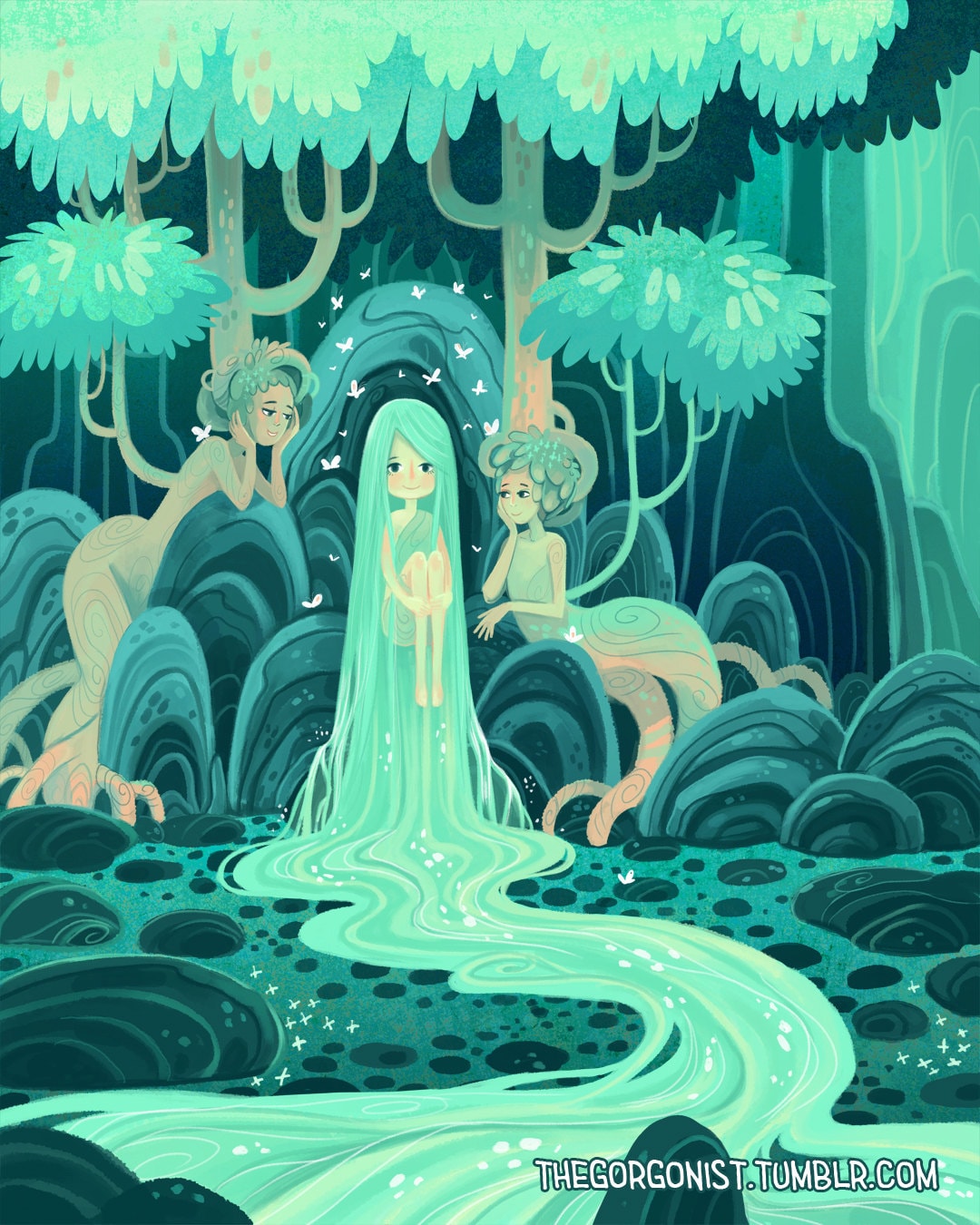This detailed fantasy illustration is bathed in an array of green hues, from dark and medium to bright and electric green. Dominating the scene is a young girl with extraordinarily long, light green hair that flows like a river, extending all the way past her feet and blending into a stream. She is seated in a fetal position, floating in mid-air and smiling warmly at the viewer. Flanking her are two ethereal women whose bodies and hair are intertwined with nature; their hair appears to be composed of leaves and plants, while their legs resemble tree trunks or roots. These figures blend seamlessly into a lush forest backdrop filled with verdant trees, bushes, and darker green rocks. Scattered around the central figure are delicate butterflies or dragonflies, their white wings standing out against the greenery. The entire image exudes a whimsical, otherworldly charm. At the bottom right corner, the text "thegorgonist.tumblr.com" is elegantly inscribed in white.